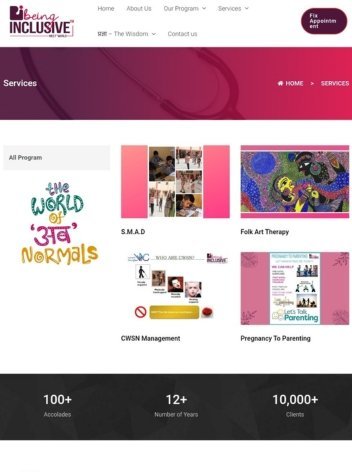The webpage features a logo in the upper left corner, difficult to decipher but appearing as either "R.I. being inclusive" or "B.I. being inclusive," rendered in shades of maroonish purple. Adjacent to the logo, a top navigation menu includes links labeled "Home," "About Us," "Our Program," "Services," "The Wisdom," and "Contact Us," some with drop-down arrows indicating additional options.

Below this header, there's a gradient box transitioning from purple to maroonish pink, with a faint stethoscope image embedded in the background. The top left of this section features the "Services" label, while the top right has a house icon followed by the word "Home," and again the "Services" label.

Further down, the content area showcases four primary boxes lined from the center rightwards:
1. **S.M.A.D.** - Features images of children.
2. **Folk Art Therapy** - Displays a piece of folk art, seemingly a painting.
3. **CWSN Management** - Includes headshots and some small, unreadable text boxes.
4. **Pregnancy to Parenting** - Shows an image of a small poster with various pieces of information.

To the far left, a light gray box reads "All Program." Below it, there's a colorful phrase stating, "The World Of [unreadable word, possibly E-F-E-T] Normals," in hues of blue, mustard yellow, and bright pinkish-purple.

At the bottom of the webpage, the footer rests on a black background, displaying:
- **100+** accompanied by "Accolades" to the left.
- **12+** with "Number Of Years" in the center.
- **10,000+** beside "Clients" to the right.